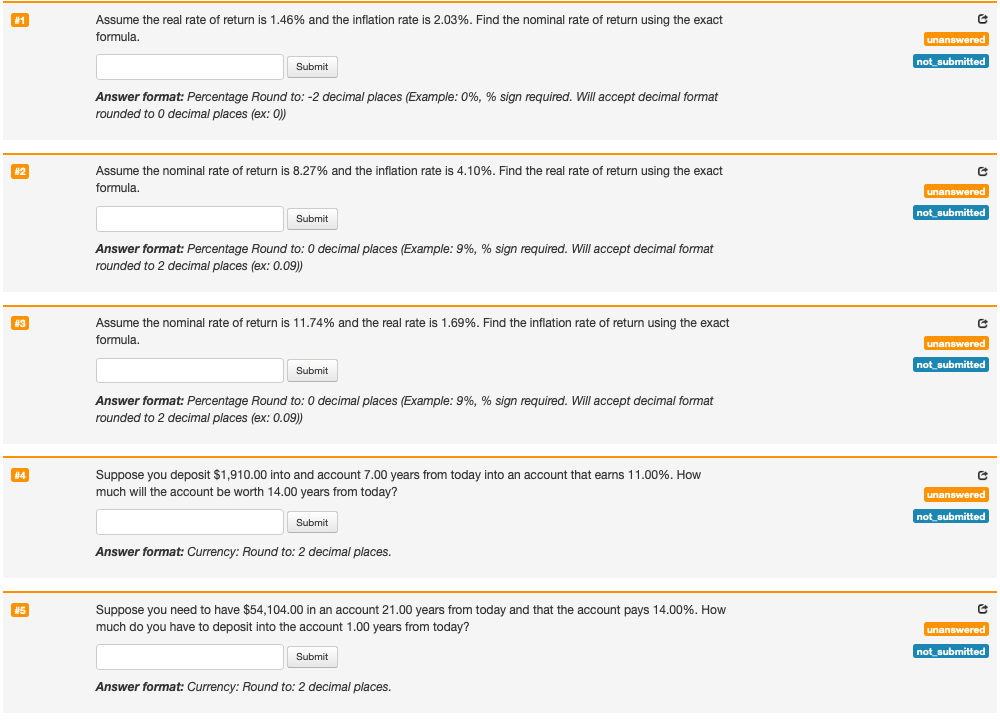A detailed square image features four distinct sections, each separated by orange horizontal lines. At the top of the image, a prominent horizontal line spans across the top section. In the top-left corner, 'Number 1' is displayed on an orange background. Progressing downward, each subsequent section is labeled sequentially as 'Number 2,' 'Number 3,' 'Number 4,' and 'Number 5.'

To the right of 'Number 1,' the text reads: "Assume the real rate of return is 1.4% and the inflation rate is 2.03%. Find the national rate of return using the exact formula." Below this instruction is a text box for input and a submit button adjacent to it. Annotations specify the required answer format: a percentage to two decimal places, with examples such as "0%." It further clarifies that a percent sign is mandatory and decimal formats are accepted, rounded to zero decimal places.

All other sections follow a similar layout, with slightly varied percentage values relevant to their respective problems. Each section has a status indicator on the right. In the first section, it says "Unanswered" in orange, with the text "Not submitted" directly below it. This pattern repeats for each section, with indicators showing "Answered, not submitted," "Unanswered, not submitted," and other relevant statuses.

Above the 'Unanswered' indicators, small boxes with arrows pointing to the right provide additional navigational cues.